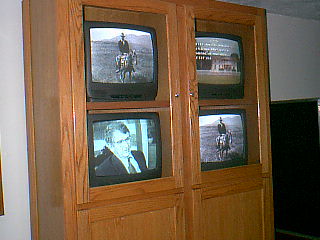The image depicts a grainy, older photograph showcasing a large, thick wooden cabinet positioned against a white wall. The cabinet, resembling an old-fashioned TV stand or entertainment center, features two sections with glass doors, through which four small, black and white televisions are visible. Each television fits into its own designated spot on two shelves. The TVs are all turned on, displaying distinct yet somewhat blurred black and white images.

In the upper left and lower right TVs, a repetitive image of a man on a horse is visible. The man and horse image is grainy and lacks fine detail. Another TV screen shows a man in a suit, who appears to be a politician, glancing to the side as if being interviewed. The remaining TV, located in the top right, shows a building with some text overlaying the image. The televisions each appear to be around 12 inches tall. This vintage setup, combined with the portrayal of repetitive and varied imagery across the different screens, lends the scene an intriguing, nostalgic atmosphere.